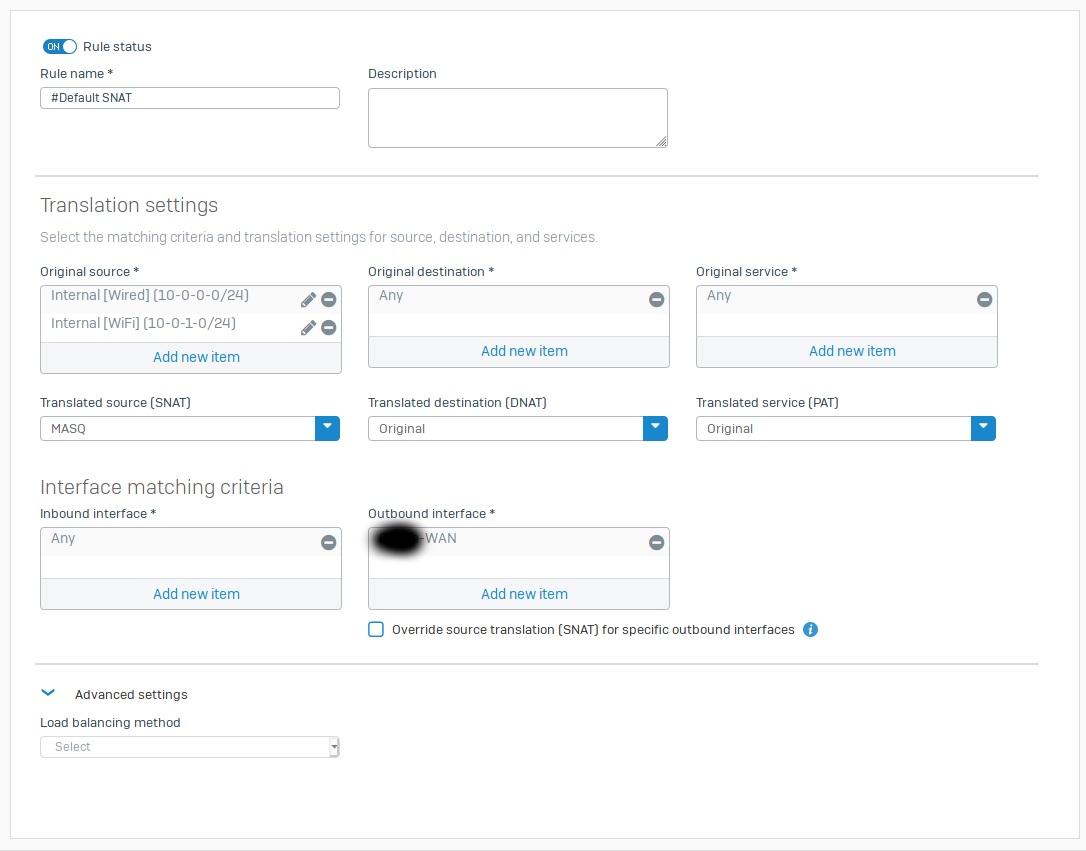A detailed screenshot appears on the screen, presumably taken from a computer or smart device, providing an internal view of selection options and settings. The interface consists of a large square with a light gray thick border and a thinner, dark gray or black inner border framing a white background similar to the standard white seen on computer screens.

In the top left corner, there's a small toggle button, which turns blue when activated, labeled "ON" in black lettering beside the text "Rule Status." Below this, in a long, skinny rectangular box, the rule name "#default_snat" is displayed. Adjacent to this is a larger rectangular box labeled "Description," which currently contains no text.

Separating the next section is a horizontal line. Below this, the text instructs users to "Select the matching criteria and translation settings for Source, Destination, and Services." 

The options are displayed in three columns titled "Original Source," "Original Destination," and "Original Service," each written in black. Below each title is a rectangular, rounded selection box containing various words and icons. A blue "Add New Item" button is available at the bottom of each column.

Underneath these columns are additional options for translation:
- "Translated Source (SNAT)"
- "Translated Destination (DNAT)"
- "Translated Service (PAT)"

Each of these also features blue arrows that can be clicked to view and choose alternative options.

Further down, users can find options for "Interface Matching Criteria," with sections for "Inbound Interface" and "Outbound Interface." Notably, the box under "Outbound Interface" has a small black smudge on it. Similar to the sections above, users can add new items here.

Additional configurable options include a button labeled "Override Source Translation." Near the bottom of the interface, there are sections for "Advanced Settings" and "Load Balancing Method."